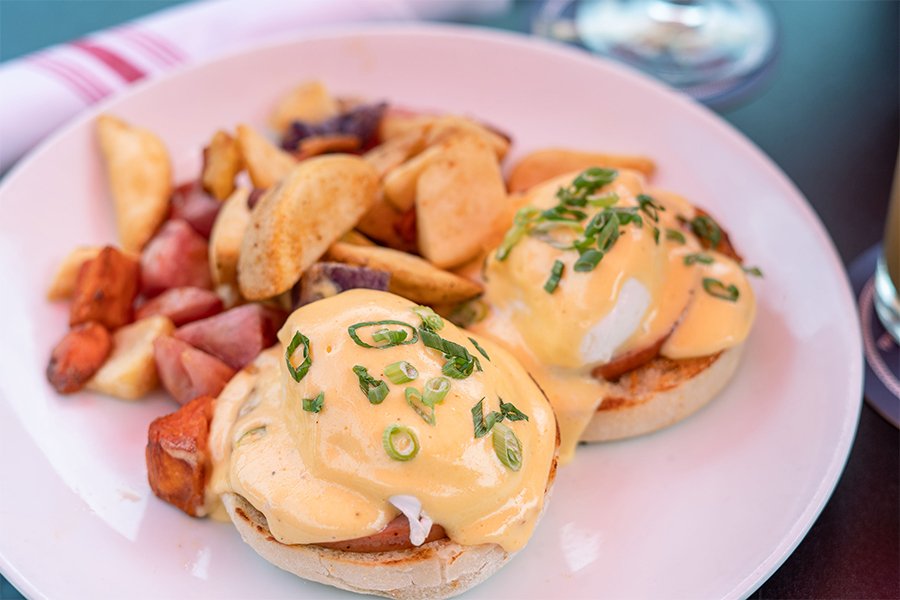This image depicts a meal served on a pink plate. At the center of the plate are two English muffins topped with poached eggs, draped in a rich, yellowish-orange hollandaise sauce that drips enticingly over the edges. Finely sliced green chives garnish the eggs, adding a pop of color. To the side, there is a portion of potato wedges, crispy and golden-brown, and some slices of pinkish meat, possibly ham or bacon. The background includes a rolled pink napkin embellished with darker pink and almost reddish stripes, as well as wrapped silverware and the base of a glass. The edges of the plate are clear, framing the meticulously arranged meal.